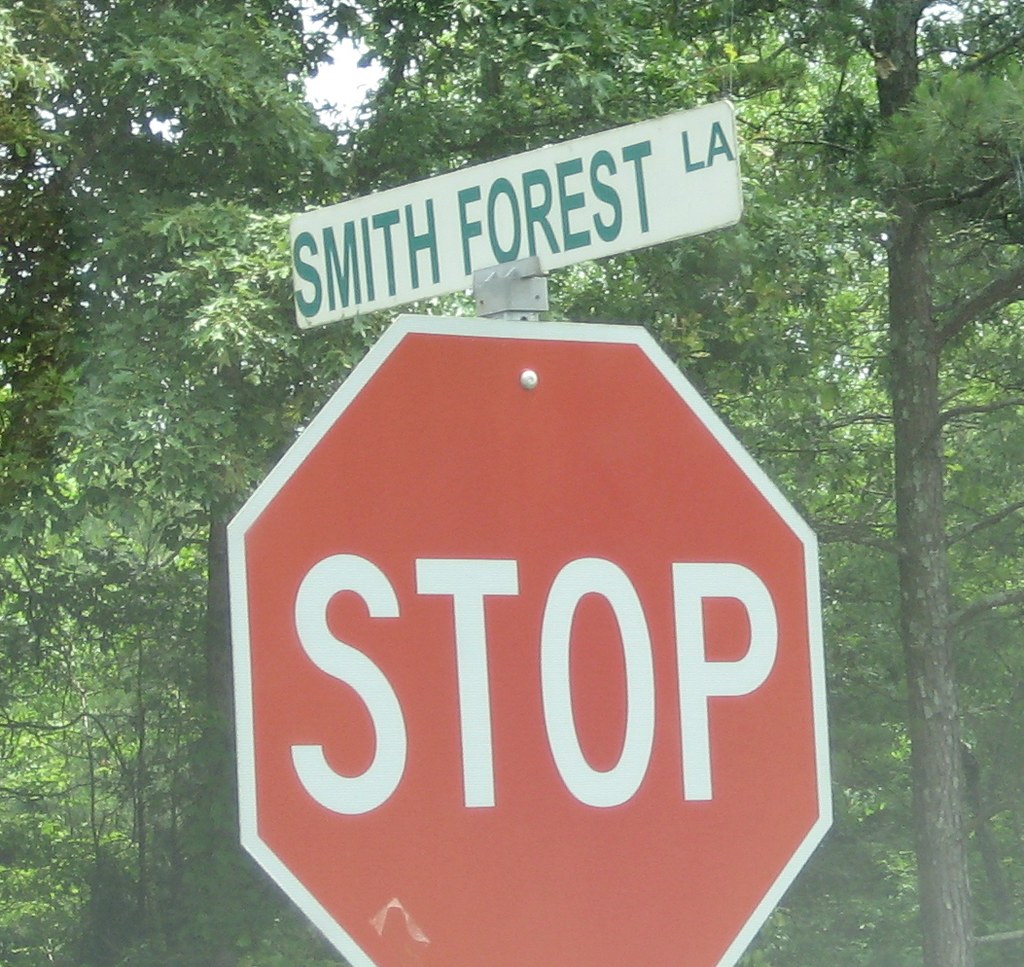In this close-up photograph, the focal point is a prominent red octagon-shaped stop sign with a white border and the word "STOP" in bold white capital letters. Positioned above the stop sign is a white rectangular street sign with green lettering that reads "Smith Forest LA," presumably indicating Smith Forest Lane. The entire scene is set against a lush backdrop of green trees and dense foliage, with a hint of sunlight peeking through in the upper left side of the frame. The image appears slightly hazy, as though taken through a slightly dirty windshield, adding a soft focus to the otherwise clear and scenic view. The stop sign dominates the center of the photograph, suggesting its placement near a road intersection.